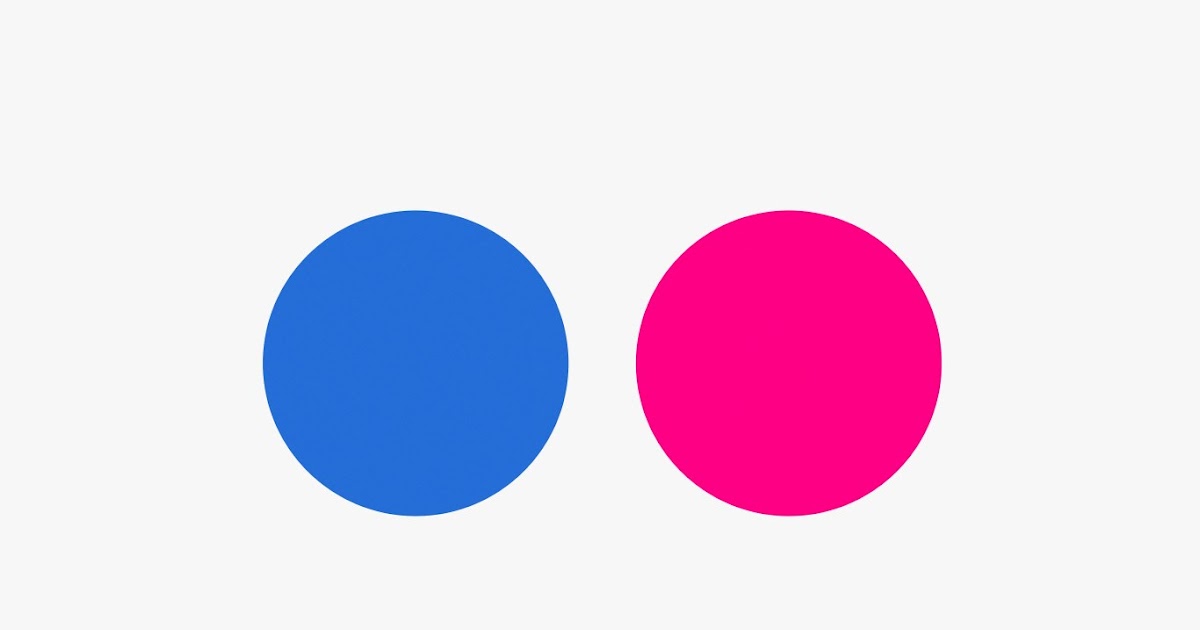The image is a minimalist design featuring a horizontally oriented rectangular canvas with a subtle, almost imperceptible gradient that shifts between very light gray and extremely light blue. Positioned on the left side of the canvas is a perfectly circular shape, filled with a solid blue color. Mirroring this, towards the right-hand side, is an identical circle in size and shape, but filled with a vivid reddish-pink hue, reminiscent of fuchsia. Both circles are precisely aligned to be at the same height, placed slightly lower than the vertical center of the rectangle, leaving more space above them than below. The circles are also equidistant from the left and right edges of the rectangle, ensuring perfect horizontal symmetry. The overall composition is striking in its simplicity, devoid of any text, figures, or additional objects, drawing attention solely to the two contrasting colored circles against the barely noticeable background.